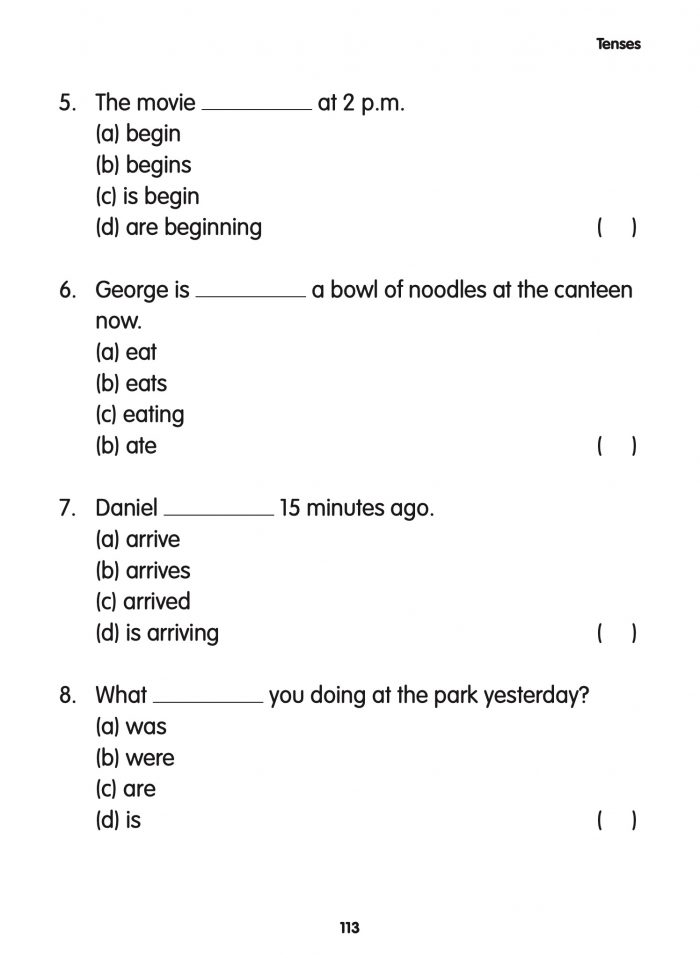This image depicts a section of a multiple-choice test or educational game, specifically focusing on questions number 5 through 8. Each question tests the participant's understanding of verb tenses. The answer choices for each question—A, B, C, and D—are listed vertically on the left side.

At the top, Question 5 reads: "The movie ___ at 2 p.m." The options provided (A) begin, (B) begins, (C) is begin, and (D) are beginning indicate that "begins" (B) is the correct answer. This question tests the present simple tense.

Question 6 states: "George is ___ a bowl of noodles at the canteen now." The choices are (A) eat, (B) eats, (C) eating, and (D) eaten, with "eating" (C) being correct. This tests the present continuous tense.

Question 7 asks: "Daniel ___ 15 minutes ago." The options are (A) arrive, (B) arrives, (C) arrived, and (D) arriving. The correct answer is "arrived" (C), testing the past simple tense.

Question 8 reads: "What ___ you doing at the park yesterday?" The choices (A) was, (B) were, (C) are, and (D) is, point to "were" (B) as the right answer. This focuses on the past continuous tense.

In the top right corner of the image, the word "tenses" is prominently displayed, indicating the central theme of this test section.